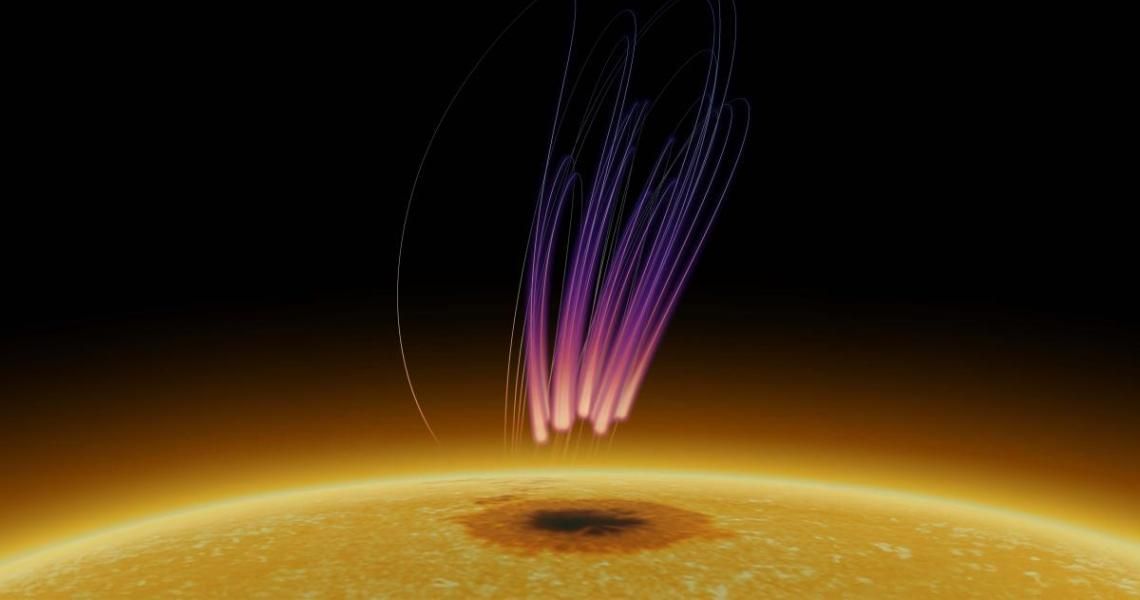The image is a digitally rendered, artistic depiction of the sun. Dominating the scene is a large, curved section of the sun, glowing in bright orange and light yellow against a stark black background. The edge of the curvature is vividly highlighted, resembling neon light. At the center of this curvature, there is a prominent burnt orange circle with a dark black splotch in its middle. Radiating from this black center are numerous thick, neon-purple lines that gradually thin out into single tendrils as they extend outward, resembling the tapered legs of a jellyfish. These lines transition from a vibrant neon pink to a deeper purple before finally vanishing into the surrounding darkness. Scattered across the sun's orange surface are small white specks, giving the appearance of being dinged. The rectangular composition of the image emphasizes the dramatic contrasts and detailed textures, creating a striking visual representation of a celestial event.